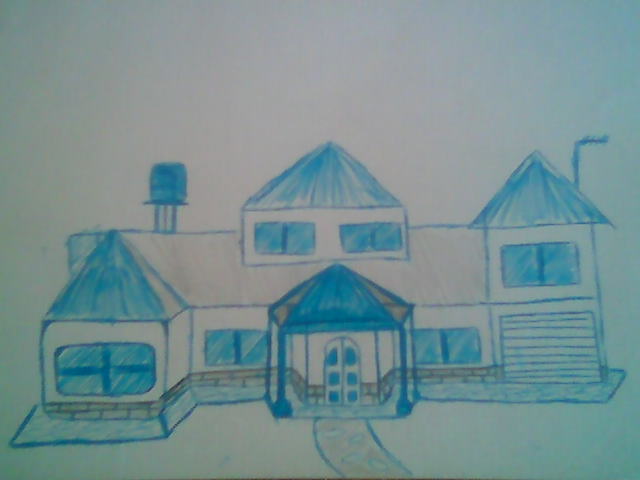This illustration depicts a charming house, meticulously colored with pencil and crayon. The vibrant scene features a front portico and a well-defined sidewalk that wraps around the entire property, providing a welcoming pathway from the bottom of the image. The sidewalk itself is detailed with shades of orange and accented with blue rocks, which are thoughtfully outlined in blue.

The house boasts several distinct architectural features. On the right side, there is a garage door with horizontal panels, topped with a horizontally sliding window. This section of the house has a peaked roof, from which a pipe extends upward and then turns to the right. The main section of the house features a brown roof, with an additional structure rising from it, adorned with two side-to-side sliding windows and topped with a blue peaked roof.

To the left, towards the back, there is what appears to be a raised structure resembling a water tower, capped in solid blue, complete with a circular platform. Additionally, a left-side bump-out features a blue window with four bars and is crowned by a peaked roof.

The front entrance is equally detailed, with a blue roof over the portico, black brick accents around the base, an arched doorway with double doors, and matching windows flanking the entrance. The entire drawing exudes a quaint, cozy atmosphere, brought to life with a rich palette of colors and intricate design elements.